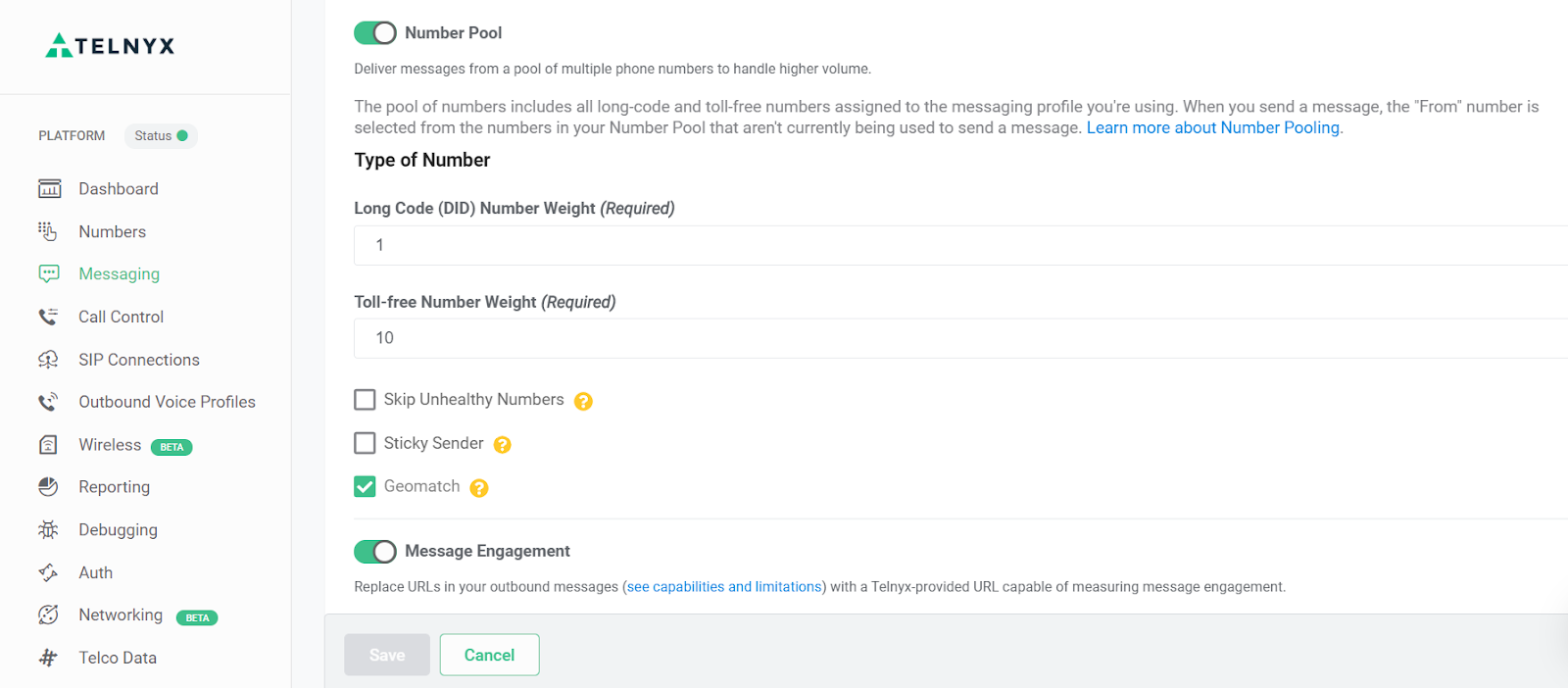This is a detailed screenshot of the Telnyx platform interface. In the upper left-hand corner, the Telnyx logo is displayed—a triangle composed of three green sections. Below this, there is a vertical menu on the left side of the screen with various navigation options, each accompanied by a representative icon. The options listed are: "Platform," "Status" (indicated with a green circle icon), "Dashboard," "Numbers," "Messaging," "Call Control," "SIP Connections," "Outbound Voice Profiles," "Wireless" (marked as "BETA"), "Reporting," "Debugging," "Auth Networking" (also marked as "BETA"), and "Telco Data."

In the main section of the interface, there is a prominent header labeled "Number Pool" with an enabled toggle switch next to it. The details below include fields and settings such as “Type of Number,” which is specified as "Long Code," "DID," and "Number Weight Required." Although the specific functionalities are not entirely clear, these terms seem to relate to phone number configurations. At the bottom of the page, another toggle switch is visible, also enabled, labeled "Message Engagement."